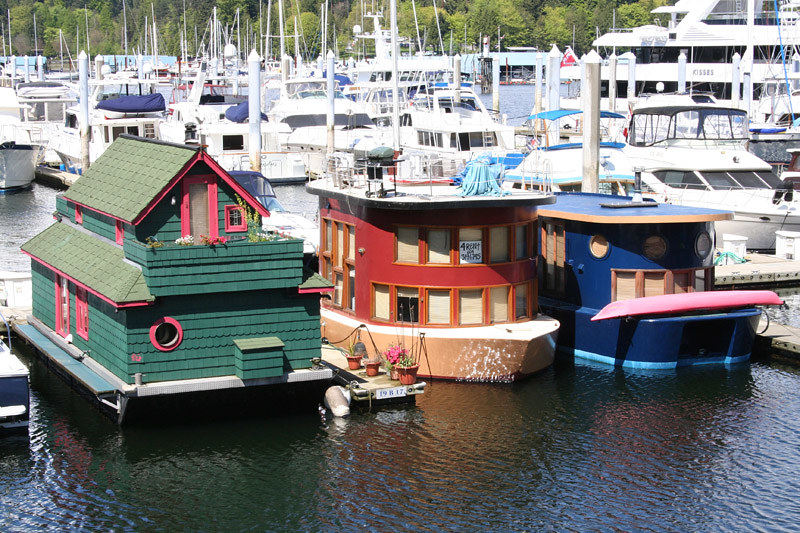The image displays a vibrant and bustling marina under the shining sun, showcasing an assortment of boats, including sailboats and yachts, in the background. Dominating the foreground are three distinctive houseboats, moored side by side. Each houseboat is unique in color and design, adding character to the scene.

The houseboat on the left is painted in a rich green with striking hot pink trim around its round window, door, and window frames. This two-story vessel features wood shingles in varying shades of green and boasts flower boxes brimming with blossoms on the upper floor, lending it a homey and inviting appearance.

The central houseboat is a warm red with orange-tinted window frames. Emblazoned with the word "For Rent," it also includes a phone number beneath the sign. A lighter tan and white section on the lower part of this boat adds contrast. Sunlight filters through partially drawn blinds, with one shade notably pulled up, hinting at the activity within. On the top deck, a barbecue grill suggests leisure and relaxation.

To the right is the navy royal blue houseboat, adorned with brown wooden trim and featuring distinctive round windows. A pink canoe is prominently draped across its front, potentially stored for future adventures on the water. This colorful ensemble is complemented by pots of flowers arranged on the dock between the boats, enhancing the scene's lively and picturesque ambiance.